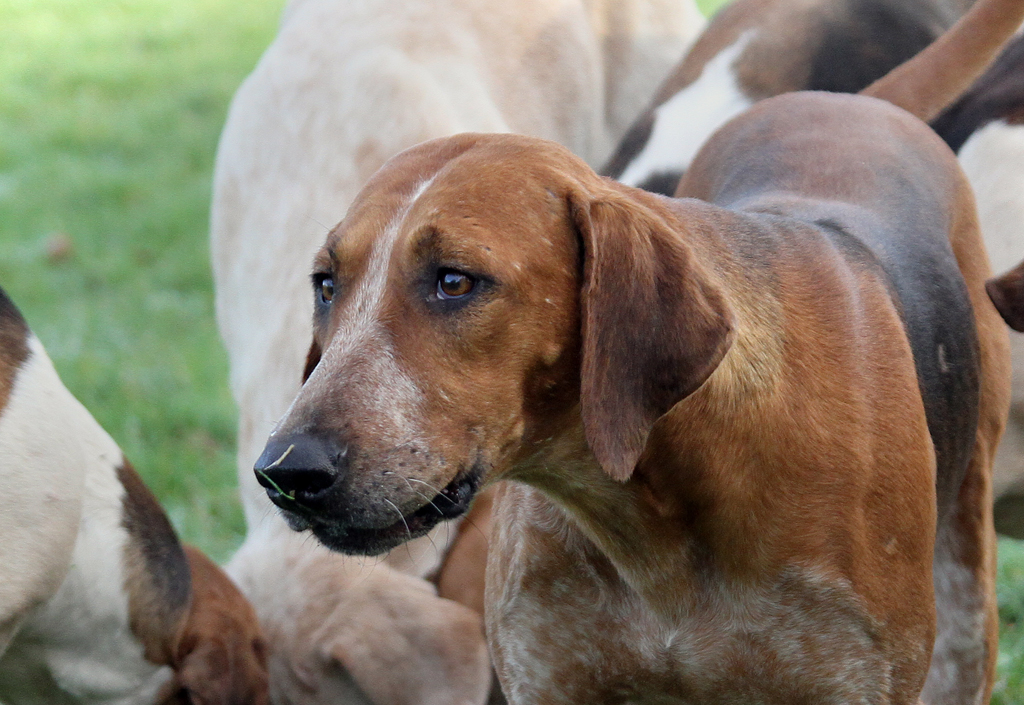The picture showcases a group of dogs in a green, blurry field, with the main focus on a distinguished beagle mix. This central dog, with a brown body accented by black markings, sports a white streak extending from its nose over its head. It gazes off into the distance, mouth partially open as if chewing or preparing to bark, with a piece of grass attached to its nose, suggesting recent sniffing activity. Its expressive brown eyes and floppy ears add to its character. Behind this main dog, about four other dogs are partially visible in the frame, bending down towards the ground as if sniffing or eating. A tan or yellow Labrador Retriever stands in the left third of the frame, facing the ground, while amidst them, one or two brindle-colored dogs can be seen in the far right. The combined scene creates a lively tableau of canine curiosity and interaction.